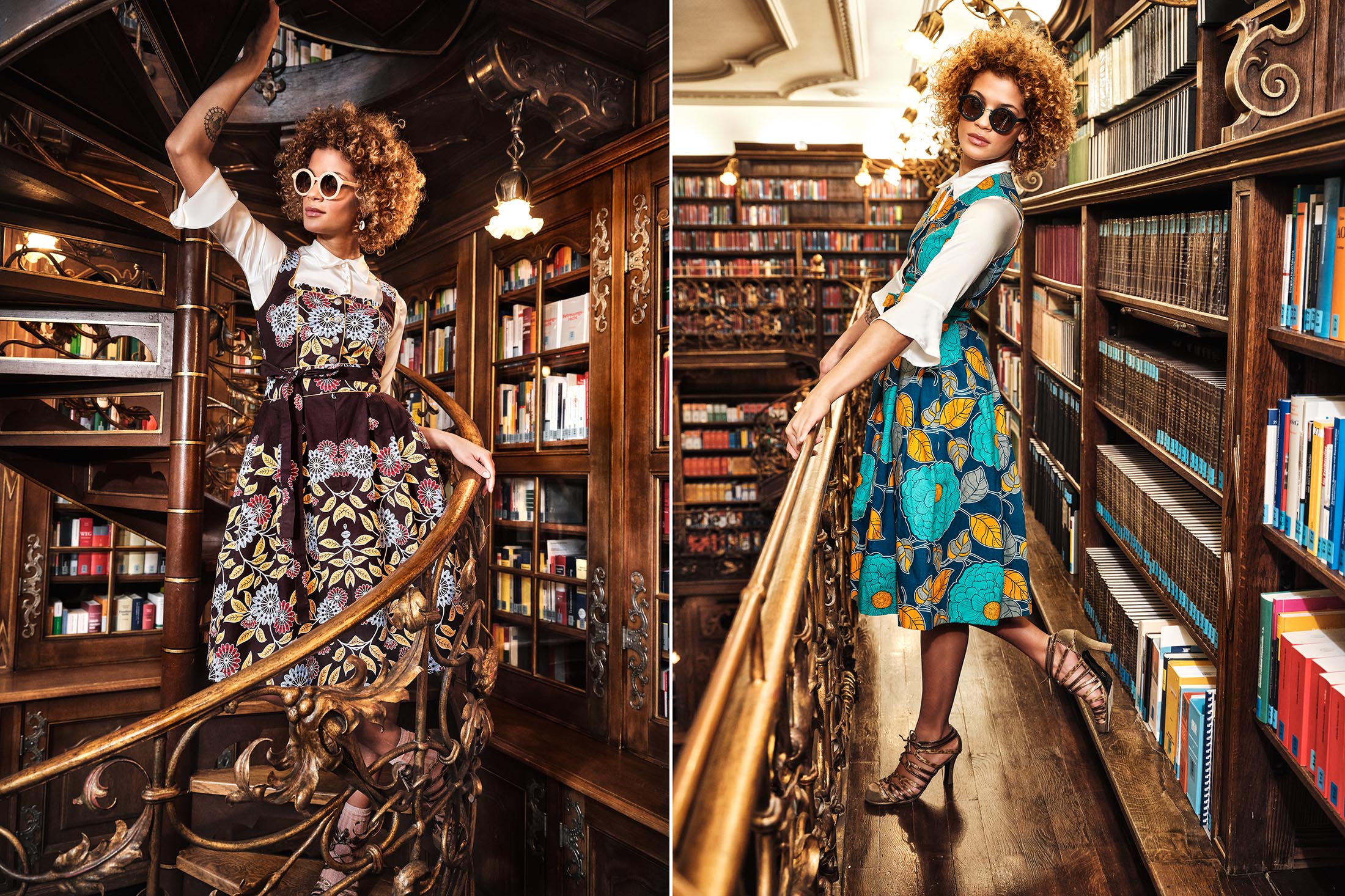The photograph collage features two images of the same woman in a library setting. In the left image, she stands on a brown wooden spiral staircase with her hand raised. She wears a white collared shirt with elbow-length sleeves, paired with a vibrant dress that has a brown fabric adorned with yellow, blue, and red foliage patterns. Her accessory choices include round white-framed sunglasses and she showcases her short, curly hair with a reddish tinge. The background features rows of bookshelves.

In the right image, the woman is depicted from the side, gazing towards the camera while holding a handrail over a balcony. She sports the same white collared shirt underneath a bright blue dress decorated with yellow, light blue, and orange leaf and flower prints. In this photo, she wears dark brown sunglasses with a distinct brown rim and high heels. The setting remains consistent with the left image, as she is again surrounded by bookshelves filled with books, underscoring the library environment.